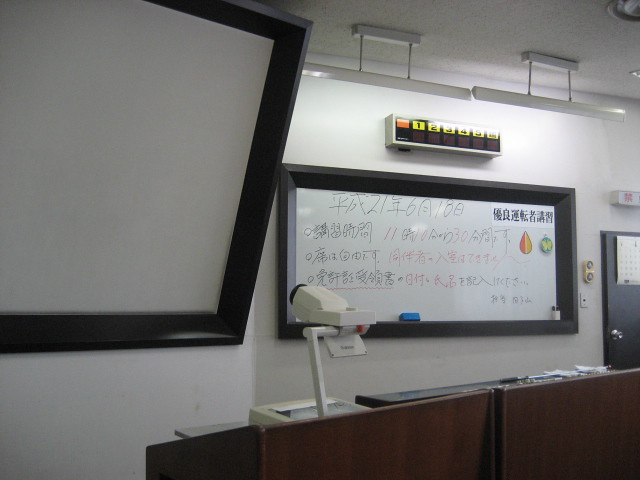This photograph captures the detailed interior of a lecture hall. At the front of the room, a large whiteboard spans the white wall, which is filled with black and red characters in what appears to be either Japanese or Chinese. Above the whiteboard, there are two pendant fluorescent lights providing ample illumination. To the left side of the image, a white overhead projector, positioned in front of a large projection screen with a black frame, is partly visible. There is also a smaller whiteboard with a thick black molding frame centered on the larger whiteboard. 

Above the whiteboard setup, a white shelf holds black boxes labeled with yellow stickers displaying numbers one through six. On the right side of the photograph, a doorway with a black door and silver handle can be seen. A light switch is mounted on the adjacent wall. The bottom portion of the image shows the top of a reddish half-wall barrier and an educator's desk. This space is clearly designed for teaching, highlighted by its thoughtful arrangement of educational tools and lighting.